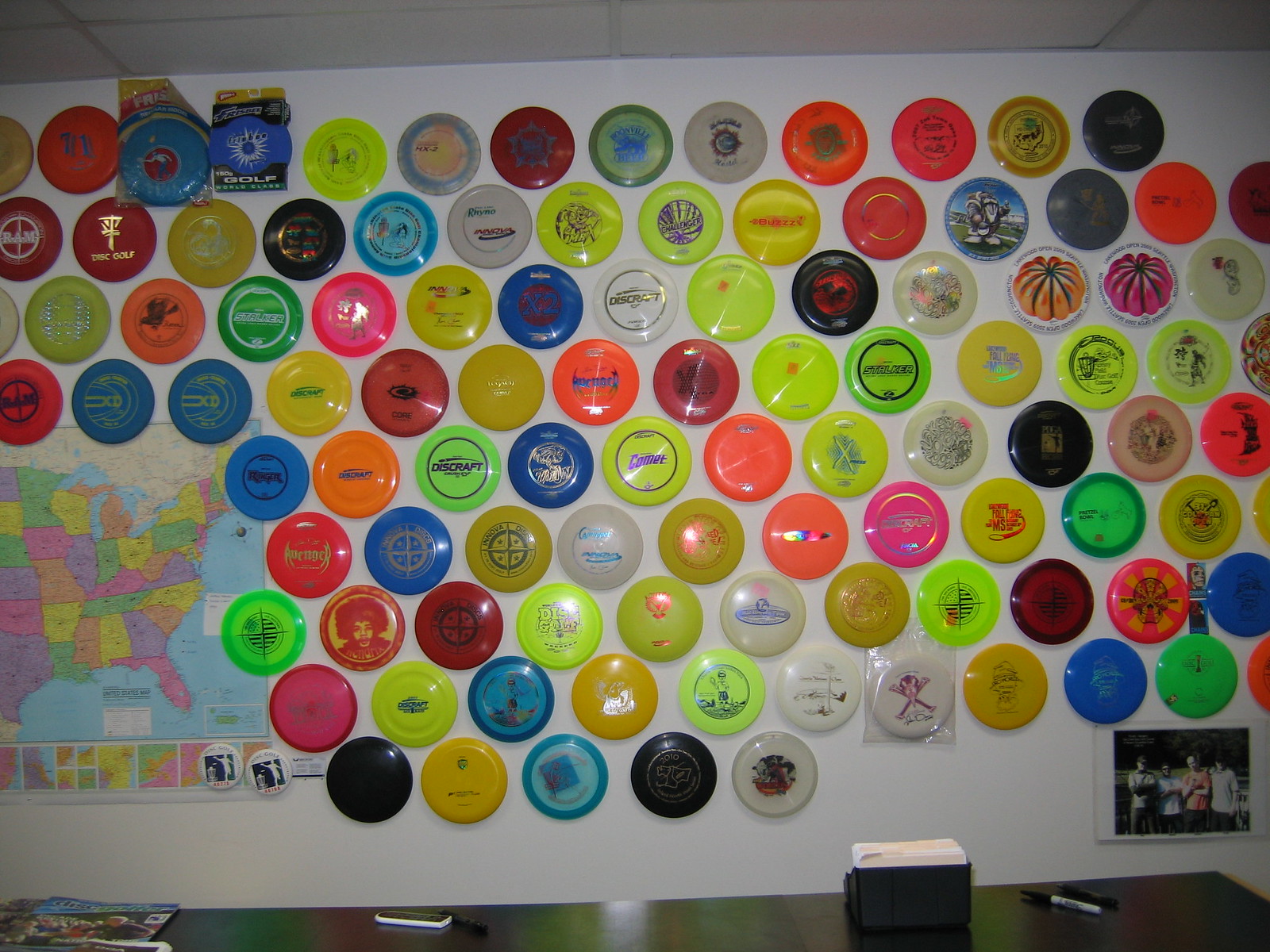This color photo depicts a white wall, possibly within a classroom, adorned with an extensive collection of multi-colored frisbees. The frisbees, which appear in colors such as neon yellow, green, orange, pink, blue, red, clear, white, black, and various multi-patterned designs, cover the majority of the wall and even extend beyond the frame of the image. Each frisbee showcases different wording, patterns, and pictures, indicating a likely passion for collecting. In the bottom left corner of the wall, there is a partially visible map of the United States, displaying the different colored states. Adjacent to this, and partially out of view in the bottom right corner, is a photograph of four young men. In front of this vibrant display rests a desk cluttered with files, papers, and markers, further suggesting a personal or perhaps educational setting.